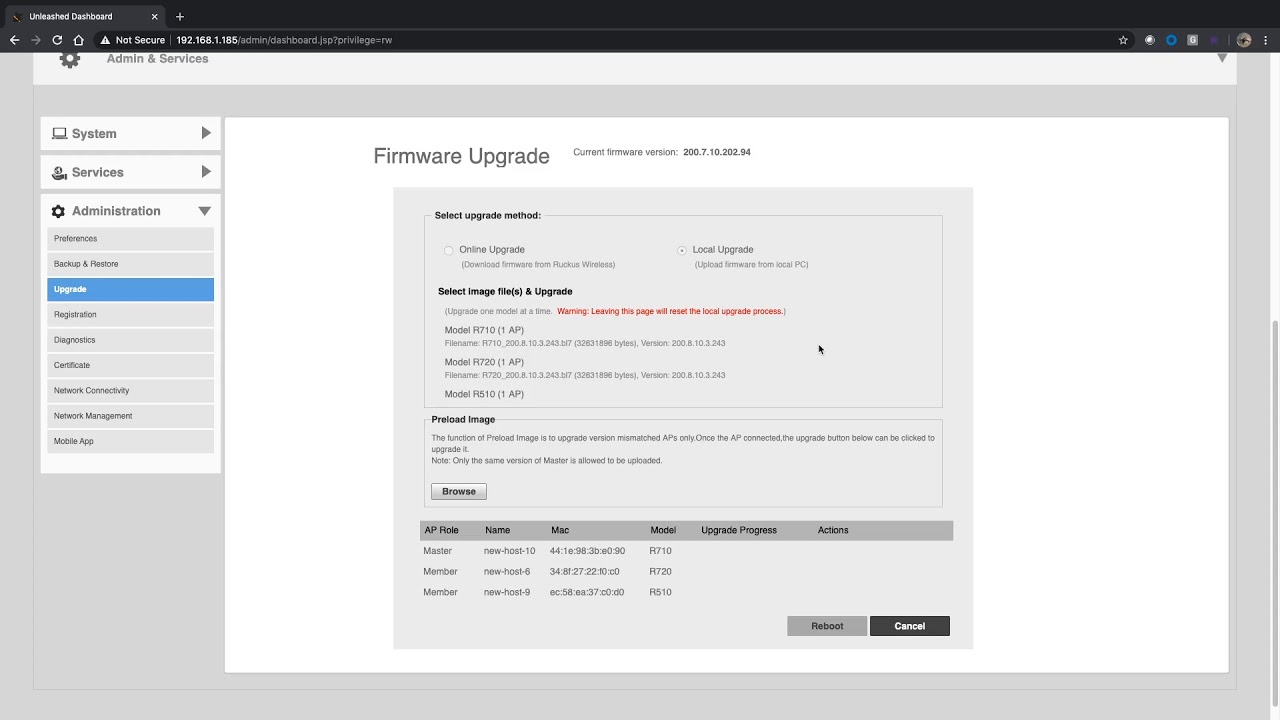In this image, we see a computer screen with a web browser open. The top section of the image, constituting roughly 10% of the screen, features a solid black background spanning from side to side, containing the website URL on the left and a single browser tab open. 

Below this, the screen transitions to a light gray background on the left side, where the words "admin" and "services" are prominently displayed. Underneath this are three categories listed vertically: "system," "services," and "administration." The "administration" category is expanded to reveal nine sub-categories in small text, with the third sub-category highlighted in blue, indicating that it is currently selected.

In the center of the image, there is a large white square background with the heading "Firmware Upgrade" written in gray text at the top. Below this heading is a light gray square area containing several sections. The first section is labeled "Select Upgrade," followed by "Select Range." The surrounding text in this section is quite small and predominantly gray, with one notable red sentence toward the top. 

Further down, there is a "Browse" button encased in its own boundary, alongside three items, each labeled within six distinctly black text categories against a gray background. At the bottom of this white area are two prominent buttons labeled "Restart" and "Cancel."

The bottom and right-hand side margins of the screen return to a gray background, framing the central content.